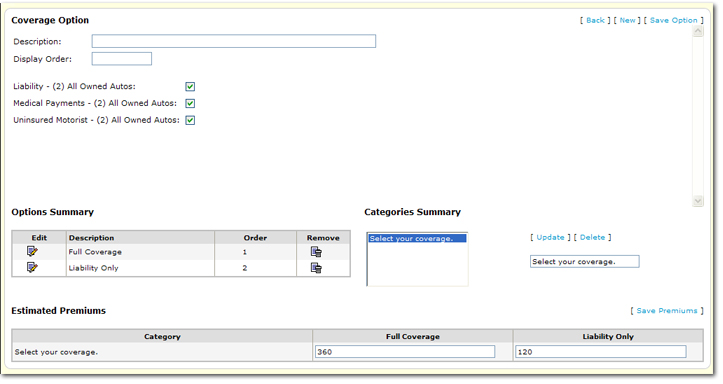This screenshot displays a user interface window for an automotive insurance coverage selection tool, likely used by insurers or their agents. The window is organized into several sections with multiple interactive elements. 

In the top right corner, there are navigation tabs labeled "Back," "New," and "Save." The top left corner identifies the window with the title "Coverage Options."

Directly below the title, there are two text boxes: one for entering a description and another for specifying the display order. Following these are three checkboxes in a vertical arrangement, each with a corresponding coverage type. The checkboxes are as follows: 
1. "Liability or Own Autos" (checked with a green tick),
2. "Medical Payments" (also checked),
3. "Uninsured Motorists" (also checked).

Further down, there are sections for summarizing coverage options and categories. These include labels such as "Option Summary," "Full Coverage," "Liability Only," and "Category Summary," accompanied by instructions to "Select Your Coverage" and estimated premium amounts. The premium estimates listed are $360 for "Full Coverage" and $120 for "Liability Only."

Overall, the layout and elements suggest that this tool assists users in selecting appropriate automotive insurance coverage, providing options and estimated costs for various coverage levels.